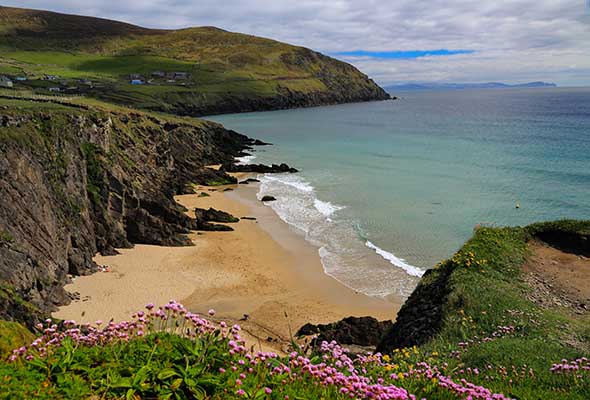This image captures a vibrant and dynamic coastal landscape, viewed from the edge of a high cliff. In the foreground, the rugged cliffside is adorned with patches of green grass and a diverse array of flowers in pink, yellow, and possibly light purple hues. The central focus is on a secluded, sandy beach nestled within a canyon-like ridge. Large rocks, apparently fallen from the surrounding cliffs, intermingle with the sand. The azure ocean waves roll gently onto the shore, creating whitecaps as they crest. 

Above the sandy beach, lush green rugged hills stretch into the distance, with their summits dotted with quaint small huts and buildings. The top left of the image reveals another cliff with more buildings perched on it, suggesting human habitation in this natural paradise. The sky above is mostly cloud-covered, though patches of blue sky peek through, adding depth and contrast to the scene. The overall setting evokes a tropical, serene ambiance with its scattered natural formations and burst of colors.